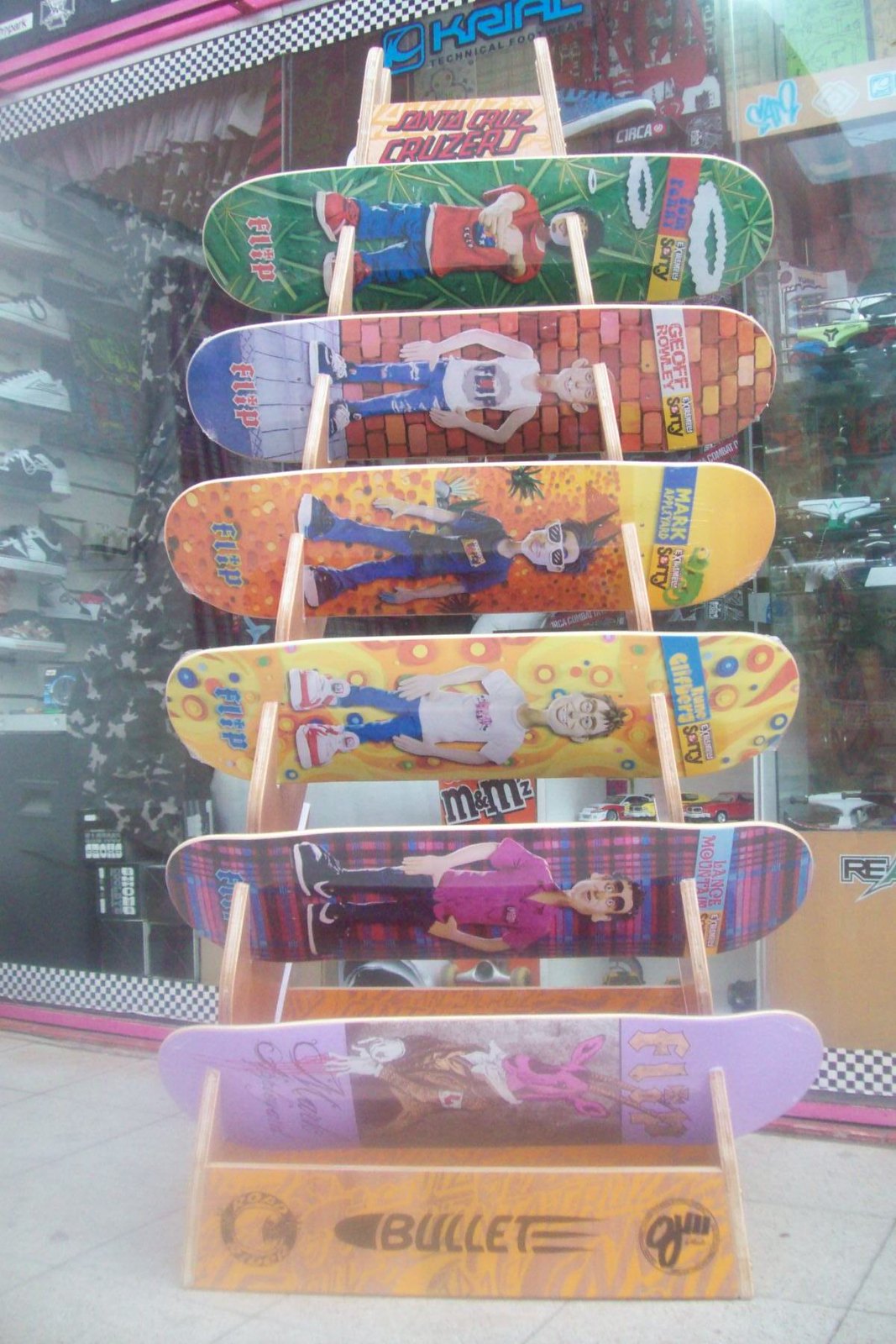This image depicts the exterior of a sports shop, easily recognizable by its window display of sneakers and tennis equipment. Dominating the scene is a tall, pyramid-like wooden rack showcasing six skateboard decks. The racks are labeled "Santa Cruz Cruisers" at the top and "Bullet" at the bottom, the latter designed as a projectile shooting left.

The skateboard decks are vividly detailed with diverse motifs and vibrant colors, each featuring cartoon-like characters in various attire. From the bottom up, the first deck is light purple, adorned with what appears to be a kangaroo or deer creature wearing a brown jacket. Above it is a blue, red, and maroon checkered board with a man in black jeans, black sneakers, and a bright pink shirt. The third deck has a yellow hue, depicting a jolly figure with red sneakers, a white t-shirt, and blue jeans. The middle deck showcases a yellow and orange theme with a character sporting spiky hair and glasses. Next is a design resembling a face brick wall with a man standing on a concrete pavement, hands on hips, dressed in a white tank top, blue jeans, and blue sneakers. The uppermost deck is overwhelmingly green, featuring a male figure in a red shirt, blue jeans, and red sneakers.

The detailed and colorful designs of the skateboard decks, combined with the distinct branding and the bustling sports shop backdrop, capture the vibrant, energetic essence of skateboarding culture.